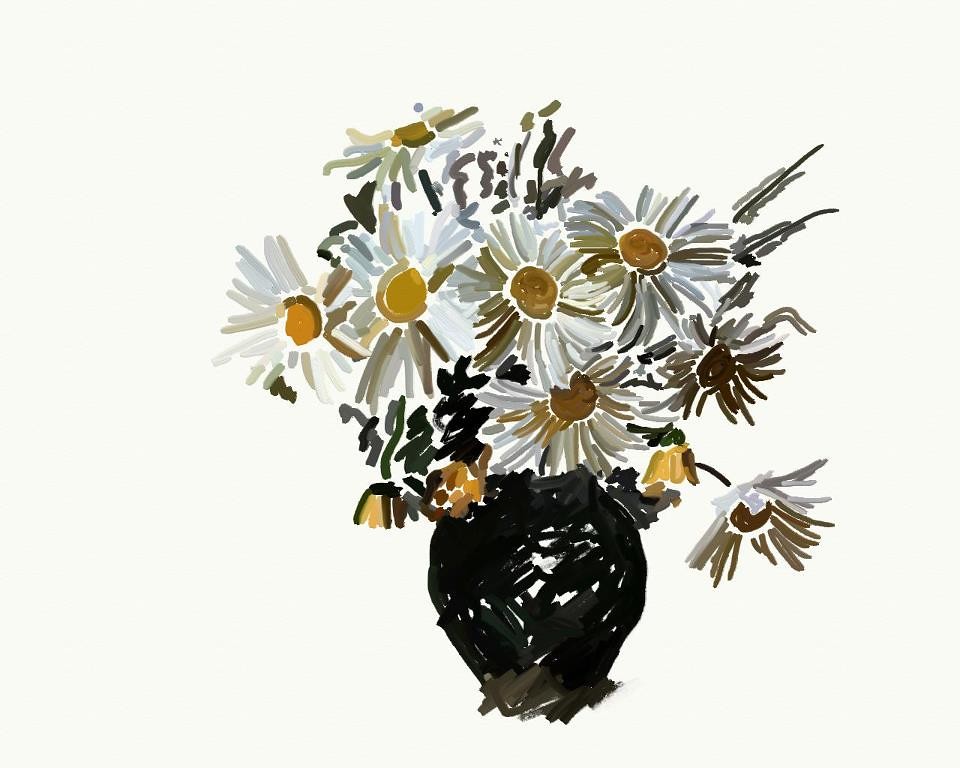A beautifully intricate drawing graces an off-white background, subtly tinged with hints of tan. The focal point is a black vase, depicted with scribbled lines that lend it a dynamic, unfinished look. The vase's base features a subtle brown hue, enhancing its hand-drawn charm. Its elegant, curvy silhouette evokes the classic shape of a ceramic planter. Sprouting from the vase are sunflower-shaped flowers, their petals rendered in delicate white with variances in their centers. The flowers on the left have bright yellow centers, while those on the right showcase deeper, brownish middles. The petals themselves are accentuated with touches of brown, gray, and green, adding depth and dimension to the composition.